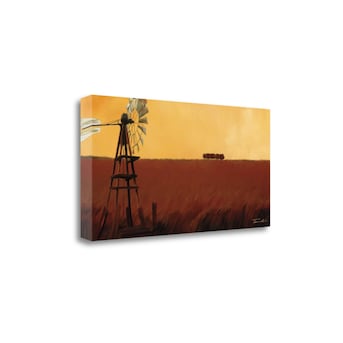The illustration features a windmill on a farm, set against a white background and tilted with its left side closer to the viewer, creating a slight 3D effect. It is presented in a landscape orientation, with the left side of the image showcasing the edge of a rectangular, thin, narrow side that continues into the visible scene. The image is divided almost evenly into two parts, with a slightly larger lower half painted in brown strokes, mimicking the appearance of a hayfield or growing wheat blowing in the wind. On the left side of the image stands an old-school windmill with a sturdy, brown and black structure, supported by four long posts and wooden brackets. The windmill's metal fan blades, which are white with a beige tint, are turned slightly towards the viewer, emphasizing their radial spokes. The background is a tan, sunset-hued sky, blending from a darker orange near the windmill to a lighter, whitish orange towards the right side of the image. A small tree line is faintly visible in the distance. The entire illustration resembles the cover of a book or a board game, adding a nostalgic touch to the agricultural scene set against the sunlit sky.